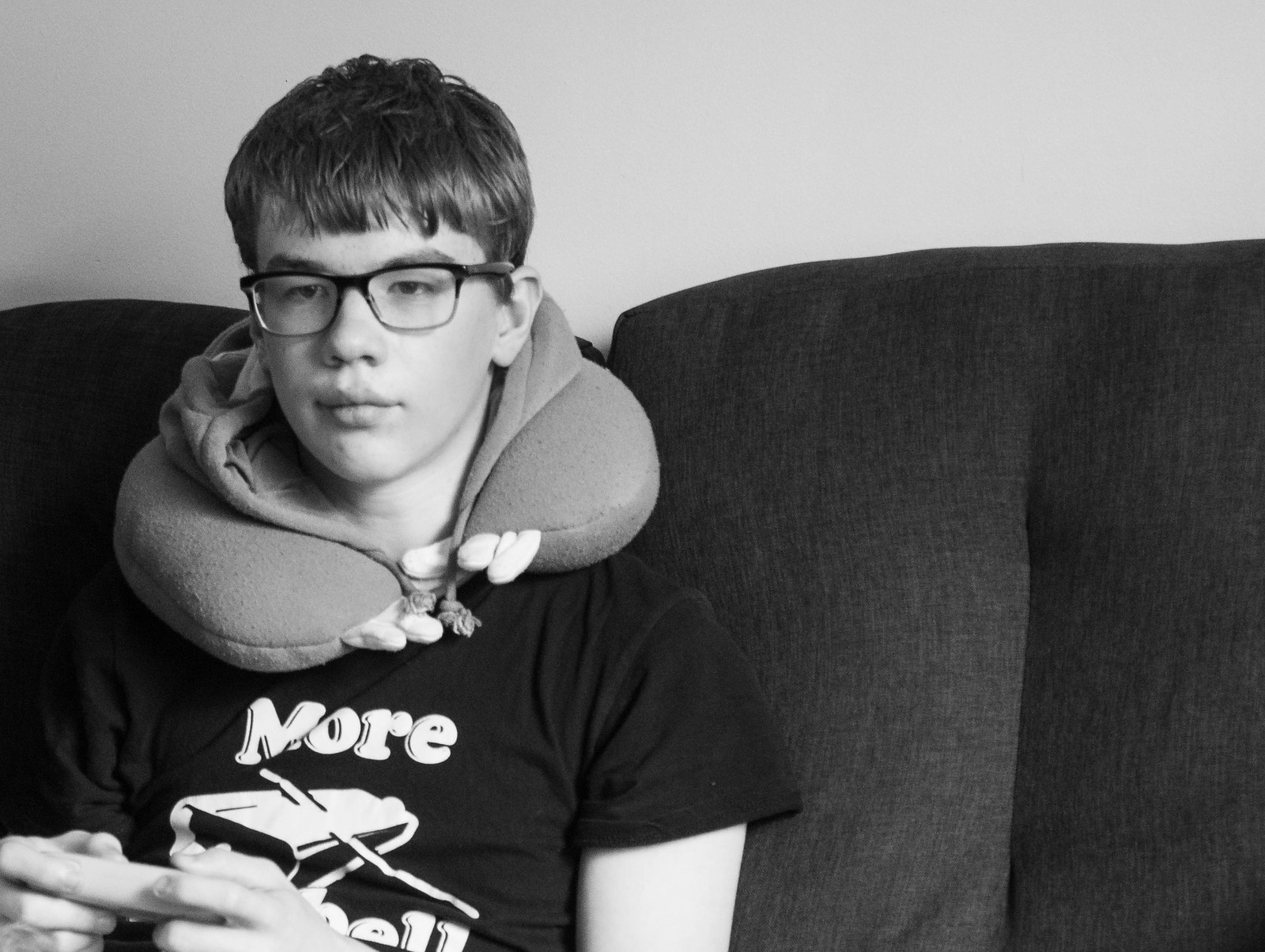This black and white photograph features an adolescent boy, possibly aged 12 to 15, intently playing a video game. Seated on a dark fabric sofa with a high back, he gazes forward with focused concentration. His short, unstyled hair and glasses frame his face, while a large, soft neck pillow, reminiscent of those used on long flights, wraps comfortably around his neck. He is wearing a black t-shirt with white lettering that partially reads "MORE" and includes an image of a cowbell, suggesting the phrase "More Cowbell." Both of his hands grip a white game controller, reinforcing his engagement with the unseen television screen in front of him. The background of the image is a plain, off-white wall, providing stark contrast to the darker elements in this monochromatic scene.